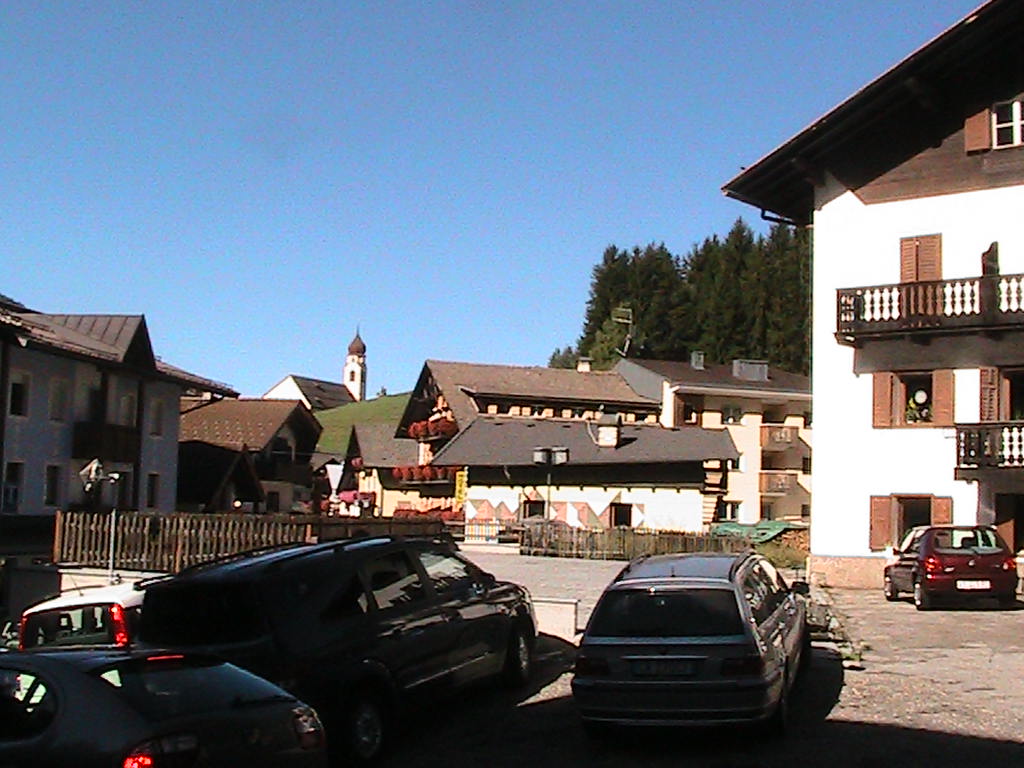The image depicts an outdoor daytime scene of a multifaceted apartment complex set against a hilly landscape. The foreground features a rectangular parking lot with several parked vehicles, including a dark gray hatchback, two vans, and a red hatchback. Some cars are shaded while others bask in sunlight. Surrounding the parking lot are multiple Bavarian-style apartment buildings, predominantly white and light brown with wood roofs, shutters, and balconies. These buildings, varying in height up to three stories, are clustered together but appear to be individual structures rather than a single complex. The upper floors show a mix of open and closed windows, hinting at the different levels of occupancy or ventilation. A notable feature is a building with an attic window ajar at the top center. 

In addition to the apartment buildings, the scenery is enriched with tall trees lining the right side, casting a natural backdrop to the modern dwellings. Green grass sweeps across parts of the hill adding a touch of nature to the man-made environment. Dominating the background, a white church steeple rises above the scene, adding a cultural texture to the landscape. The sky overhead is clear blue, completing the serene yet dynamic atmosphere of the photograph.

Overall, the image combines diverse elements including architectural styles, natural features, and everyday life in a cohesive, illustrative snapshot of a residential community.